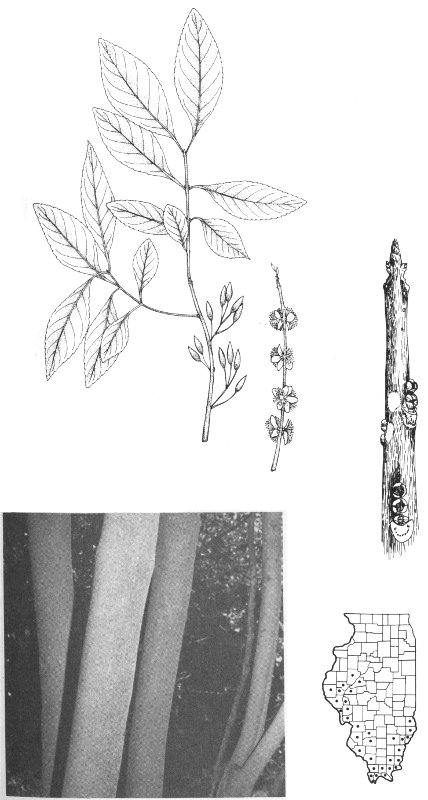This image series comprises four distinct sections against a white background, each rendered in black and white to illustrate various aspects of a tree native to Illinois. In the top left, a detailed pencil drawing showcases a vertical plant stem that branches into a leafy formation. This section also features close-up illustrations depicting additional leaves at the top and buds in different stages of growth. Directly to the right, there is a series of vertically aligned, delicate flowers.

Below these illustrations, on the bottom left, resides a black and white photograph capturing the intricate details of thin tree trunks with three to four stems emerging from the ground. Lastly, the bottom right corner presents a detailed map of Illinois, delineated by counties. Specific counties, primarily in the southern region, are marked with dots, indicating the native habitat of this particular tree species. The comprehensive combination of botanical illustrations, floral sketches, trunk photographs, and geographic mapping provides a thorough depiction of the tree's characteristics and native distribution.